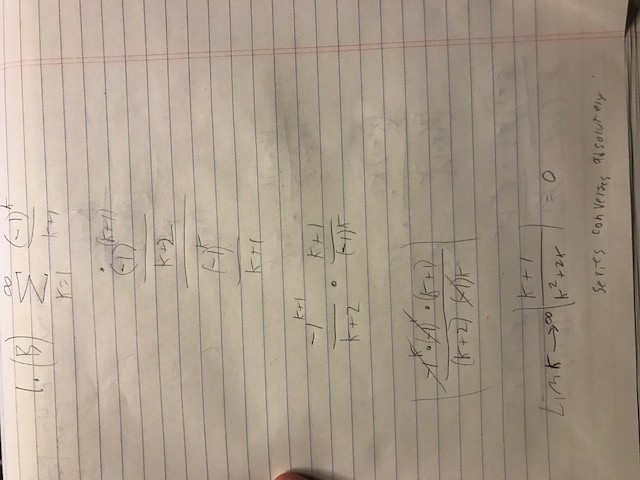This overhead photograph captures an A4-sized notepad filled with a series of handwritten equations in black biro. The page is tilted to the side, giving a unique perspective as if the image, originally taken in portrait mode, was later flipped into a landscape orientation. The equations begin on the left side of the page and progress downward, mimicking the structure of a typical written page, despite the angled view. The notepad features a series of horizontal and vertical segments of equations, starting with one horizontally written equation, followed by taller segments and groups of equations extending across the page in several rows. Towards the bottom, there is a section of smaller handwriting that is unfortunately illegible due to its size. The slightly disorienting angle and detailed mathematical notations evoke a sense of active problem-solving and intellectual engagement.